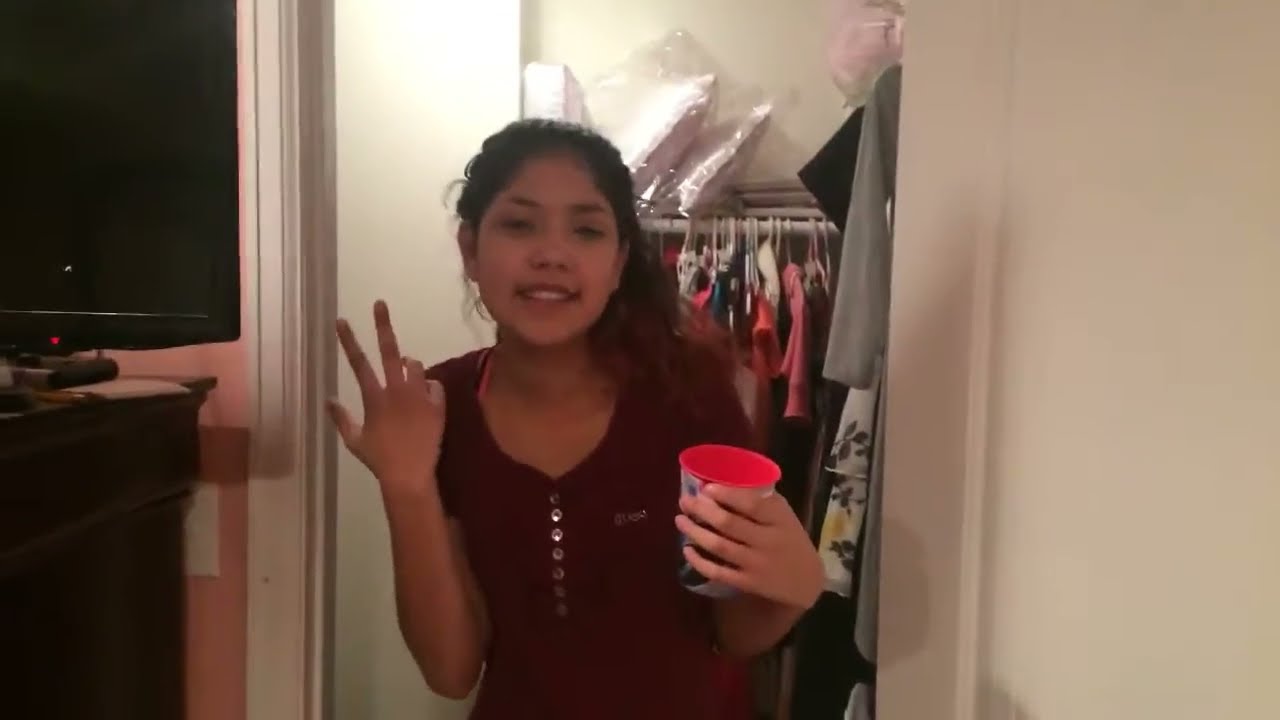In this full-color photograph taken inside a young girl's bedroom, the focal point is the girl, probably a tween, standing in the doorway of her open closet. The walls of the room are painted pink, with a door frame featuring white molding to her right. The closet behind her is brightly illuminated by an overhead light. The closet consists of a rod with multiple hangers full of clothes, and a shelf above it storing pink pillows and other items.

The girl, who has light tan skin and long dark hair cascading down her right shoulder, is wearing a short-sleeved burgundy blouse that buttons halfway down the front. She has a slight smile on her face. In her left hand, she holds a red plastic cup with a lid and white design, while her right hand is raised, displaying a peace sign with her thumb and first two fingers extended.

To the left of the girl, you can see a wooden dresser—partially visible against the pink wall—with a flat-screen TV sitting atop it.